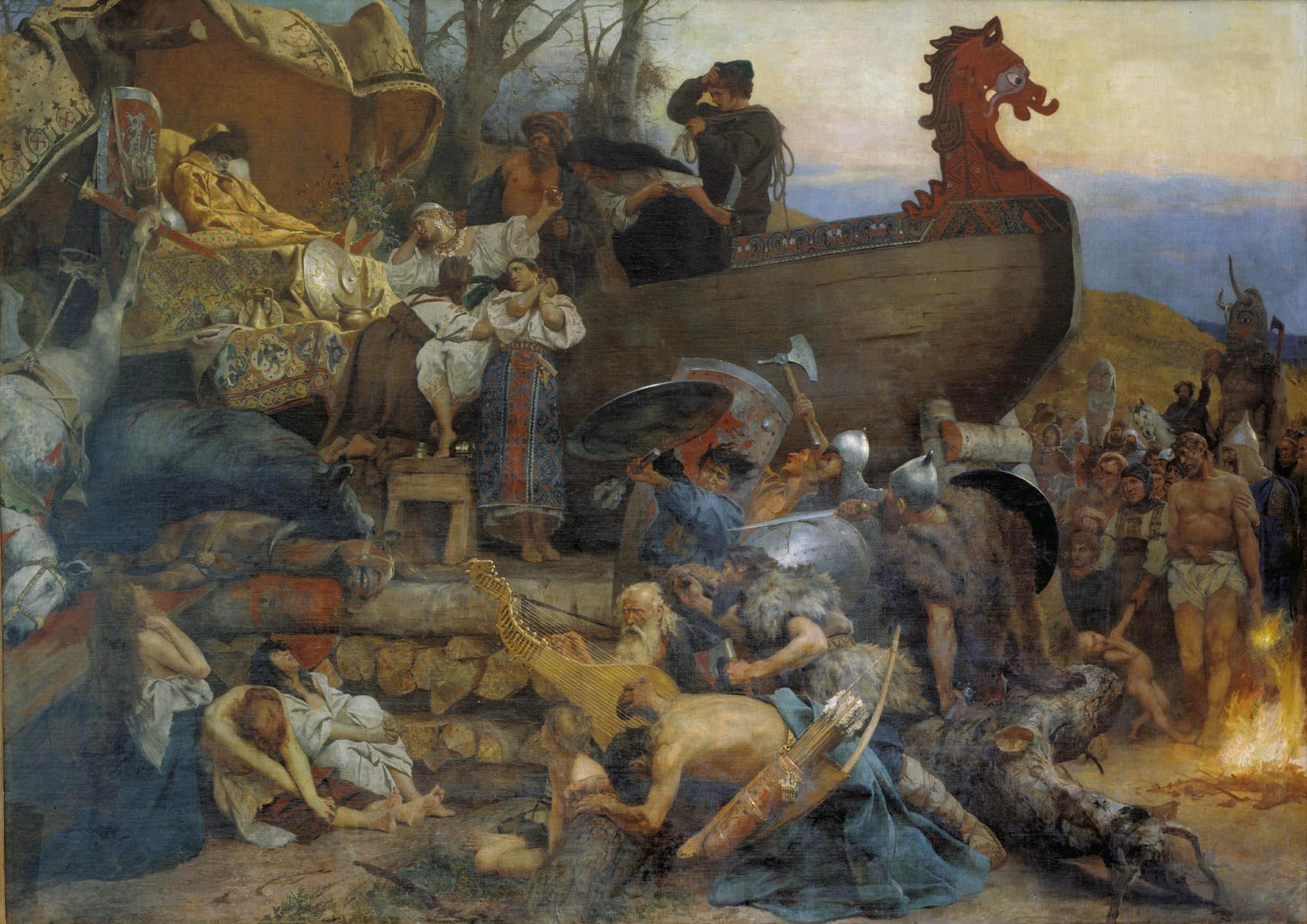This is a chaotic, detailed painting depicting a scene of apparent suffering following a ship journey, likely set around the 1500s. The grounded ship, estimated to be 35 to 40 feet long and primarily brown with a red dragon figurehead resembling an Asian dragon, dominates the scene. Surrounding the ship, a diverse crowd of nude or semi-nude people is gathered, some lying down, injured or being consoled, while others stand in various states of distress. 

Several key figures stand out: in the lower-left corner, a topless man in white shorts; in the center, an older man with a white beard playing a large stringed instrument; and nearby, a man carrying a baby. The scene also includes scattered animals and a campfire in the lower-right corner where a burning log can be seen. The painting exhibits vibrant colors, mainly blue, gold, red, and some brown.

The composition evokes a sense of a biblical tragedy, with some viewers seeing parallels to stories like Noah's Ark due to the ark-like ship and the array of suffering figures. The presence of weapons like swords and axes suggests a battle might have occurred, further adding to the image's intensity.